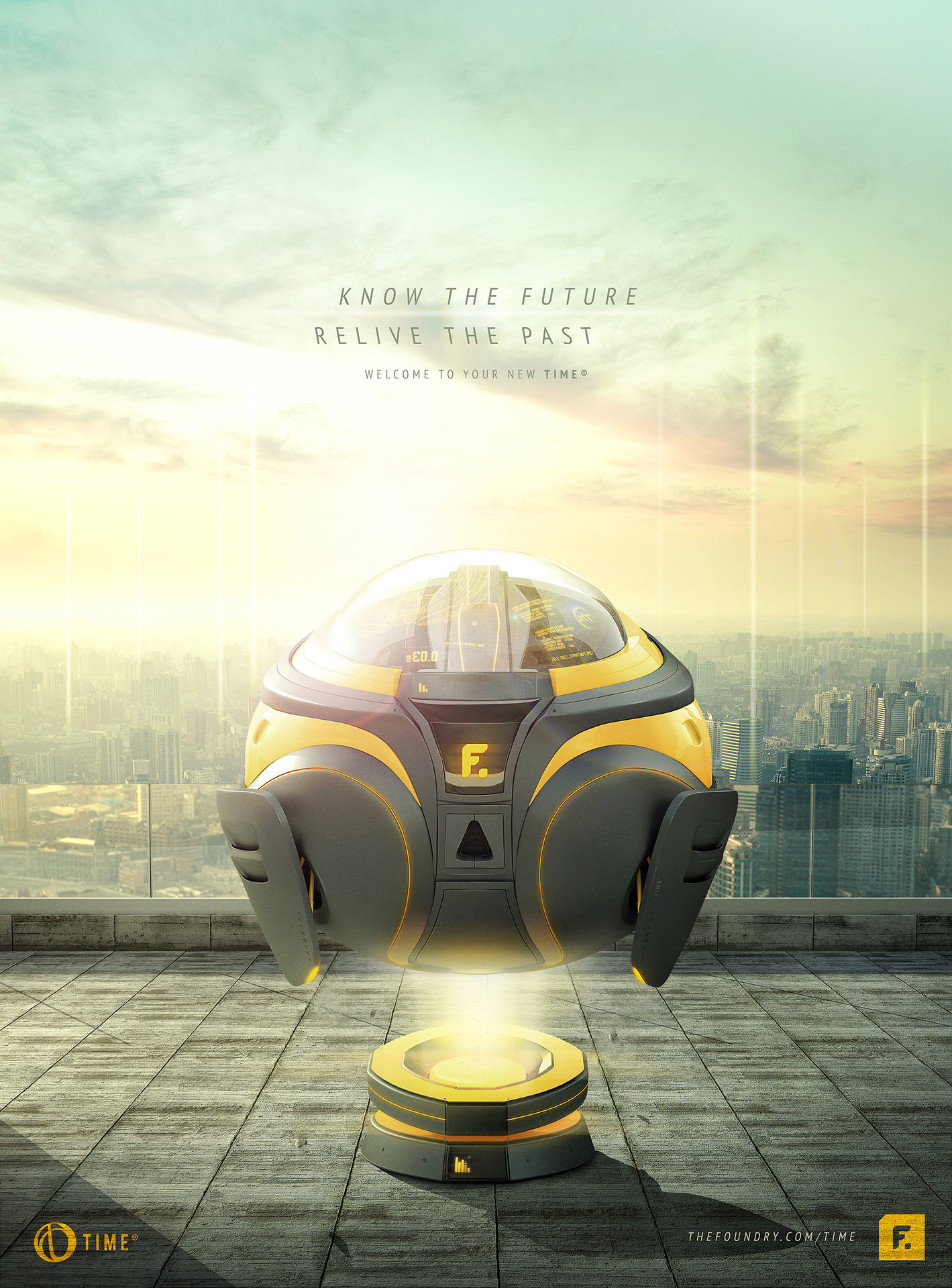This detailed poster is an advertisement that vividly depicts a futuristic science fiction scene. Central to the image is a yellow and gray rocket ship with a transparent, bubble-like dome on top, levitating just above a gray building rooftop. Emanating from the bottom of the rocket is a bright yellow light. Surrounding this focal point, an expansive city skyline stretches across the middle of the image, filled with diverse skyscrapers. The sky overhead transitions from deep blue at the top to greenish-yellow and pale yellow hues towards the center, featuring a shining sun.

At roughly one-third of the way down from the top of the poster, the text "Know the future, relive the past" is prominently displayed in dark gray, with "welcome to your new time" positioned directly below it in smaller print. Additional text is found at the bottom corners of the poster: "thefoundry.com/time" on the bottom left and a yellow "time" symbol on the bottom right. The overall design and vivid colors emphasize the futuristic theme while fitting the advertisement's style for The Foundry.